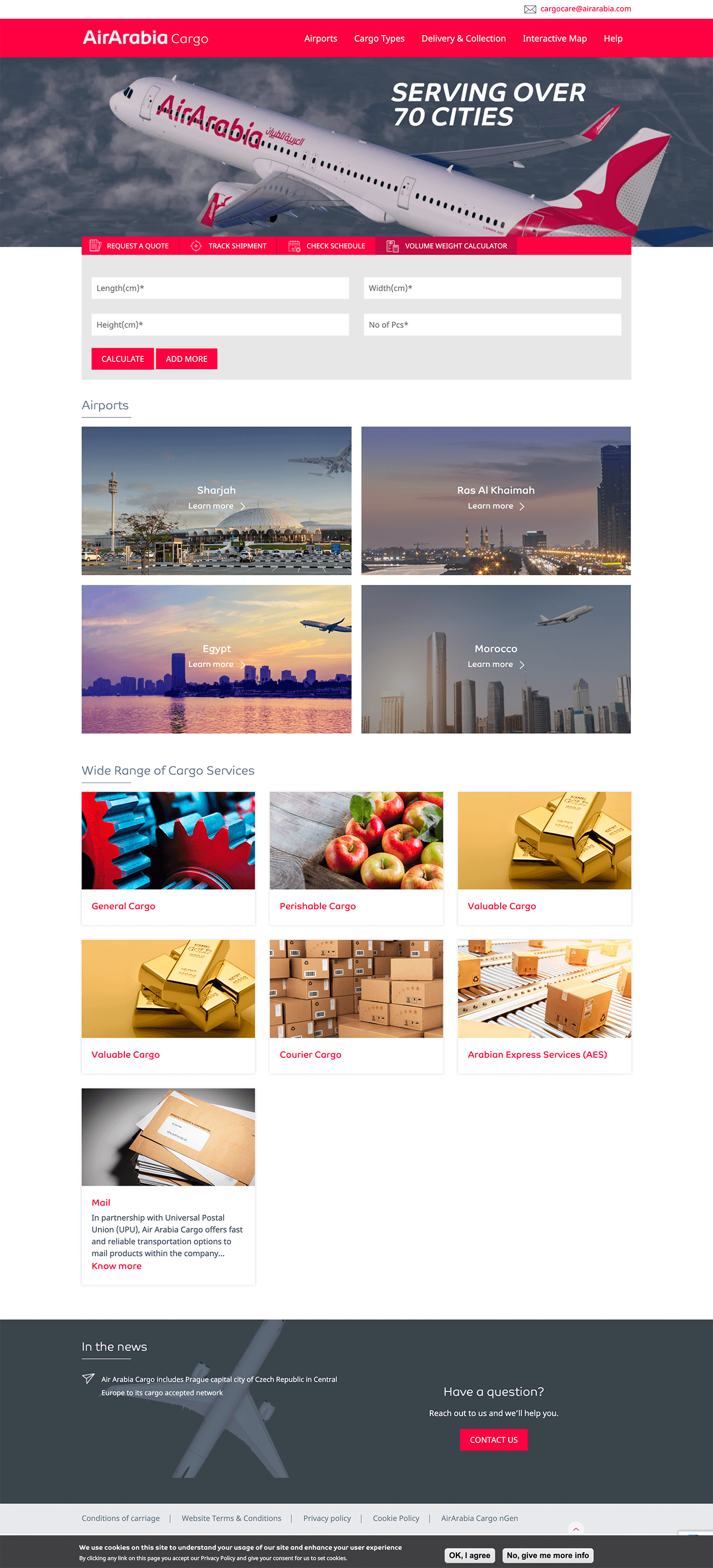This screenshot from the Air Arabia Cargo website provides comprehensive details of their cargo services. 

At the top, a red banner with white text features navigation options: Air Arabia Cargo, Airports, Cargo Types, Delivery and Collection, Interactive Map, and Help. To the top right, an envelope icon with the email "CargoCare@AirArabia.com" is displayed. Below the banner, a striking image depicts an Air Arabia airplane flying diagonally upwards to the left, adorned with the "Air Arabia" logo in red letters on its side and a red bird icon on its tail.

Beneath the image, a menu offers four key options: Request a Quote, Track Shipment, Check Schedule, and Volume Weight Calculator, with the latter being selected. The calculator includes fields for Length (cm), Height (cm), Width (cm), and Number of Pieces, along with buttons for Calculate and Add More.

Further down, sections labeled Airports, introduce Sharjah and Ras Al Khaimah airports with accompanying photographs and "Learn More" links. Another section highlights various destinations with vibrant images: Egypt, featuring a night skyline and an airplane flying in from the right; and Morocco, showcasing a city against a gray sky with an airplane ascending towards the top right.

The page promotes a wide range of cargo services. General Cargo is depicted with blue and red gears, Perishable Cargo with a crate of apples, and Valuable Cargo with gold bars. Courier Cargo is represented by stacked cardboard boxes, and Arabian Express Services (AES) by conveyor belts with boxes. Mail service is shown with a stack of envelopes and notes a partnership with the Universal Postal Union for timely mail transport.

At the bottom, a dark gray banner includes a news update about Prague joining the cargo network, a prompt for customer inquiries with a "Contact Us" button, and various policy links. A disclaimer about cookie usage concludes with options to accept or seek more information.